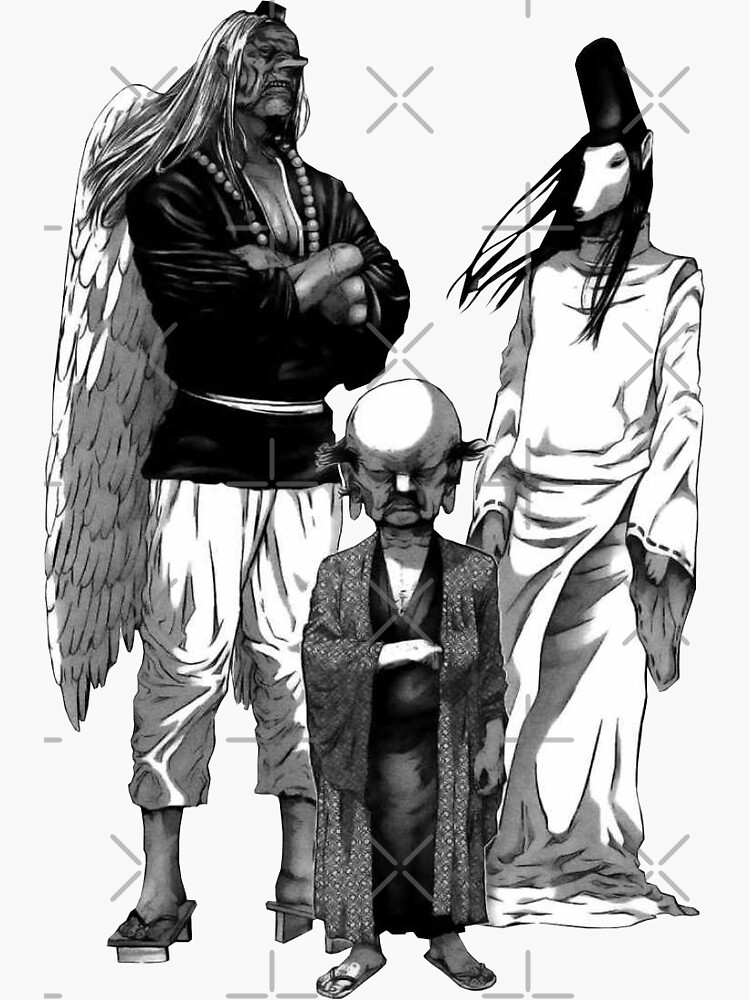The black-and-white image features three distinct humanoid creatures against a white background, each with unique characteristics. The creature on the left appears older, with a very long nose, long white hair, and pointed gritted teeth. It has white wings extending from its back and is adorned in a black long-sleeved tunic, baggy white pants, and wooden sandals. A black band is tied around its waist, and it dons a square hat atop its head. The creature on the right has the head of a dog or wolf, featuring shoulder-length black hair and wearing a white robe with long sleeves that extend past its hands. This figure's robe falls to the ground, obscuring its feet, and it sports a black hat. In the foreground, much shorter than the other two, is a creature with a rounded, bald head and hair jetting out from the sides above its ears. It is clad in an ornate patterned kimono over a black robe and sandals. The shorter figure stands slightly ahead of the other two, adding to the image's depth. The overall scene is intricate and richly detailed.